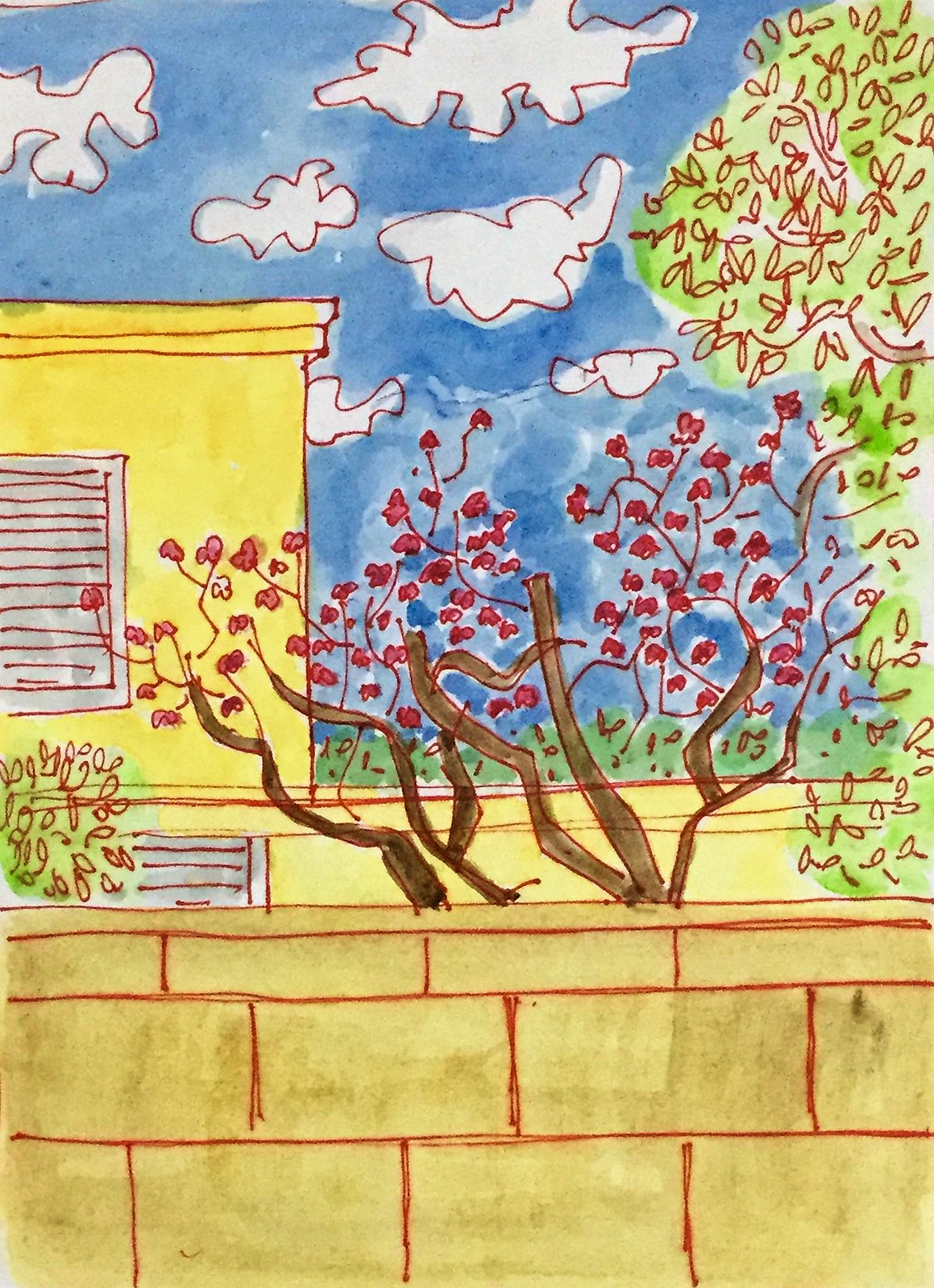This detailed watercolor and ink painting depicts a whimsical, cartoon-like scene of a yellow-brown brick or concrete block wall, distinguished by red lines that outline the bricks. The wall consists of two rows of larger blocks with smaller ones on top, and a single slab crowning the structure. Emerging from behind the wall are brown tree limbs with smaller offshoots adorned with red buds or mini-flowers, suggesting springtime cherry blossoms. On the left, a green bush sits atop the wall, while on the right, a tall tree extends upwards, its branches fanning out at the top. In the backdrop, a mustard-yellow building with distinct architectural elements is partially visible. Near the left bush, there's a gray-topped door or window with intricate line details. Another vertical section of the building rises about a quarter of the way up the image, featuring a gray window accented with red stripes. The sky above is a wash of blue, populated with whimsically painted white, puffy clouds. The overall scene is framed by a serene green background, further enhancing the playful, illustrative charm of the artwork.